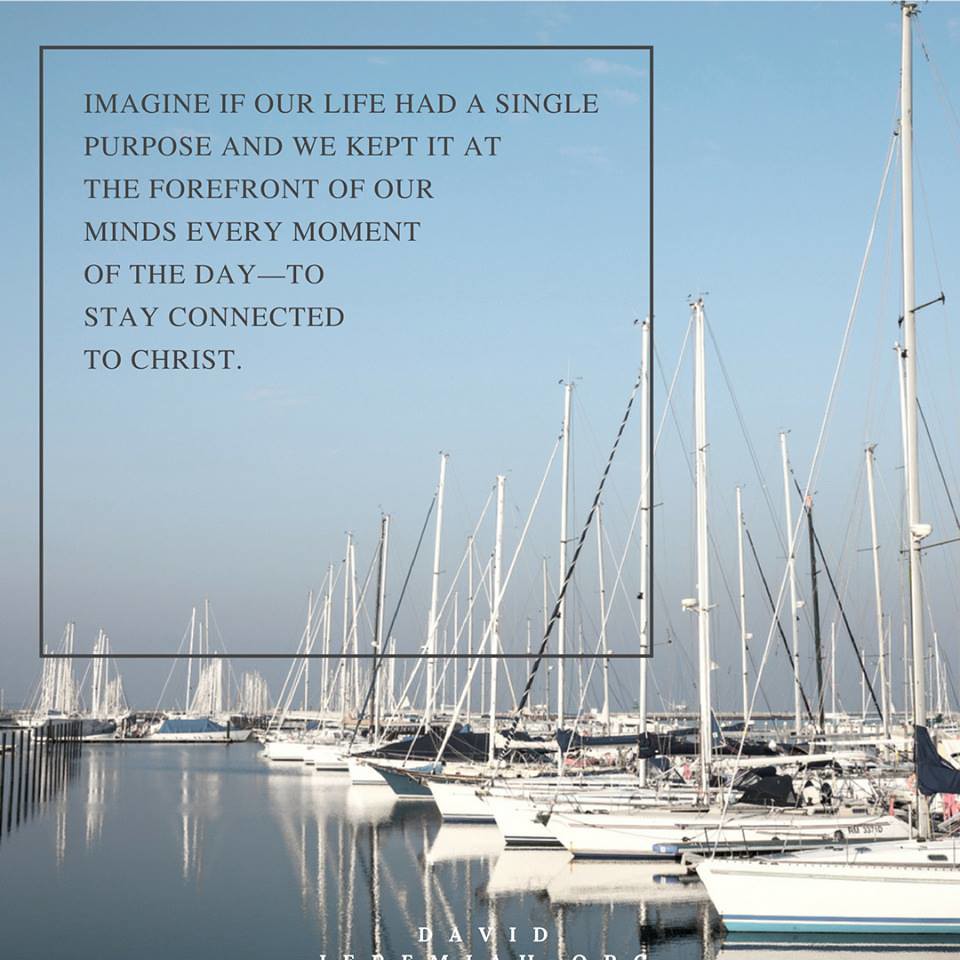In this image, a serene marina with a blue background is depicted, featuring a clear expanse of bluish water as reflective as glass. Rows of sailboats are neatly lined up, their white hulls accented with occasional black or blue stripes. Each boat's mast stands tall, forming triangle shapes, though the sails are notably absent. In the foreground, the boats are angled to the left, their bows pointing right, while those in the background recede centrally, creating a sense of depth. Overlaying the scene, a transparent square with a black outline contains the inspirational text: "Imagine if our life had a single purpose and we kept it at the forefront of our minds every moment of the day to stay connected to Christ." At the bottom of the image, centered in white text, is the partially visible name "David" followed by text that is not fully legible.